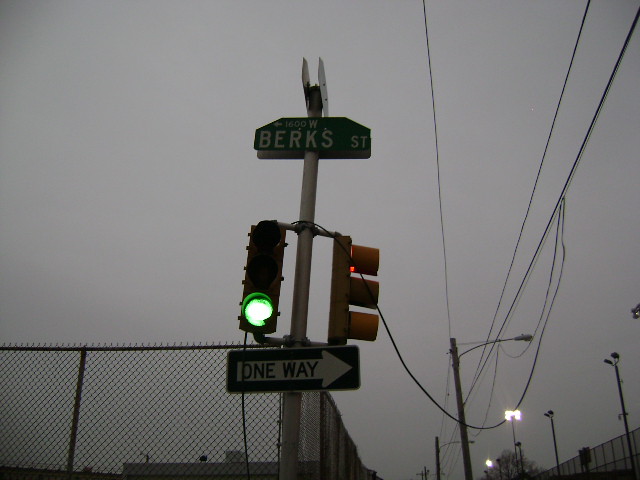This photograph, taken on a cloudy day with an overcast gray sky, captures a typical urban street scene. Dominating the center is a silver pole adorned with multiple signs and traffic lights. At the top of the pole, a green street sign reads "1600 West Berks Street" in white letters. Directly below this, a black and white trapezoidal sign indicates "600W" for West and "Berks St," with an arrow pointing to the left. Underneath the street signs, two yellow-bodied traffic lights are mounted with black metal rings. The central traffic light displays a green cylindrical light, while the other, partially obscured, shows a faint red light.

Beneath the traffic lights, a black one-way sign with a white arrow points to the right. Several crisscrossing electrical wires extend from the pole, threading through the gray sky, while more wires run towards and away from the pole, connecting to streetlights that line the unseen road. Some of these streetlights are illuminated, casting a soft glow. A dark gray chain-link fence runs along the bottom left side of the image, and another is visible on the right. In the distance, a tan building peeks over the fence, contributing to this nondescript yet detailed urban tableau.